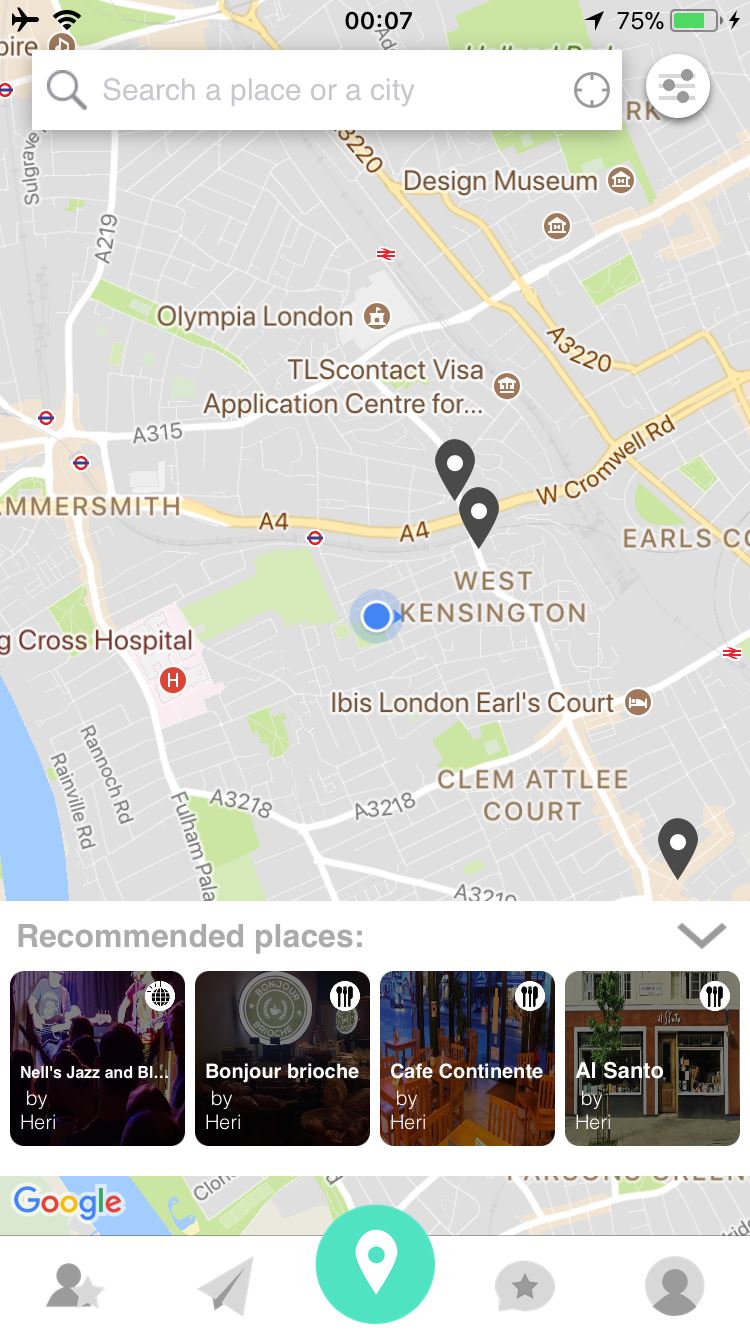Screenshot of a cell phone screen displaying a detailed map of the West Kensington area in London. The map highlights key locations such as Olympia London, the Design Museum, and the TLS Contact Visa Application Center. Various landmarks and establishments are marked, including Ibis London, Earls Court, and Clem Atlee Court. Major roads and highways are labeled, including A3-220, A3-15, A3-218, and A4 West Cromwell Road. At the bottom of the screen, several recommended places are indicated, such as Nell's Jazz & Blues, Bonjour Brioche, Cafe Continent, and El Santo, all suggested by a user or app named H.E.R.I. The interface also features multiple control buttons, including one with a person and star icon, an airplane or mail icon, a central green button with a white logo, and another silhouette icon on a green background, providing user functionality and navigation options.